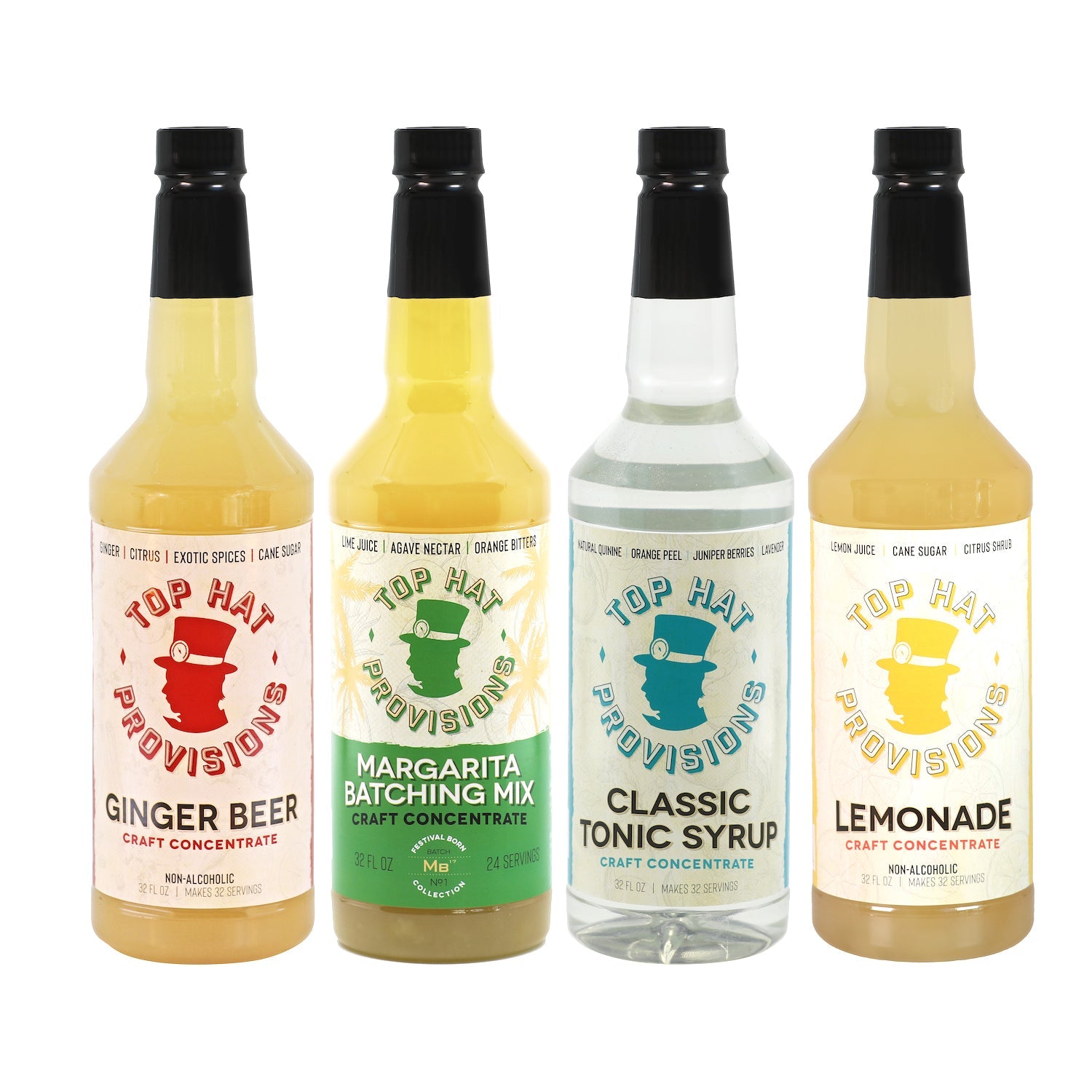The image displays four liquor bottles, each with a distinctive label and color, arranged in a row from left to right against a white background. The first bottle, containing a light yellow liquid, features the Top Hat Provisions label with an image of a person in a top hat facing left. It reads "Ginger Beer" in bold black letters and "Craft Concentrate" in smaller red font. The second bottle, also filled with a yellow liquid, has a similar label but with green elements stating "Margarita Batching Mix" and "Craft Concentrate" in black letters beneath it. The third bottle contains a clear liquid and features a blue top hat silhouette on a white label, indicating "Classic Tonic Syrup" with "Craft Concentrate" written below in smaller blue font. The final bottle on the right holds a light yellow liquid and bears a white label with a yellow top hat image. It reads "Lemonade" in bold black letters, followed by "Craft Concentrate" in smaller red font. All bottles are equipped with black twist-off caps and are uniformly sized at 32 fluid ounces. Additional minor text is present on each label but is too small to be legible.